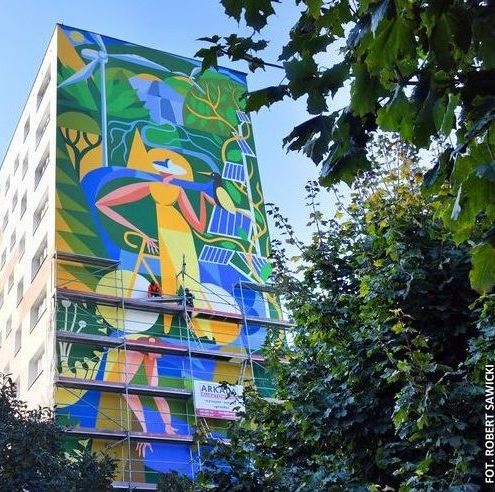The image portrays a towering building situated on the left side, isolated from other structures, and adorned with a gigantic, abstract mural that still appears to be a work in progress, as indicated by the presence of artists on scaffolds. The mural depicts a woman wearing a hat and a yellow dress, holding an exotic bird in her left hand, amidst lush foliage with a stream running through it. The scene is further animated by small solar panels encircling the woman and intertwined vines. The lower half of the building is shrouded in scaffolding, hinting at ongoing work, while a sign on the scaffolding partially reveals the name "Arcada." The bottom right corner of the mural bears the signature "F.O.T. Robert Sawicki," or "Sanwicky," though the exact spelling is unclear. The right side of the image captures some green bushes and possibly a tree, suggesting the photo was taken from a distance to encompass the entire building and its vibrant mural.